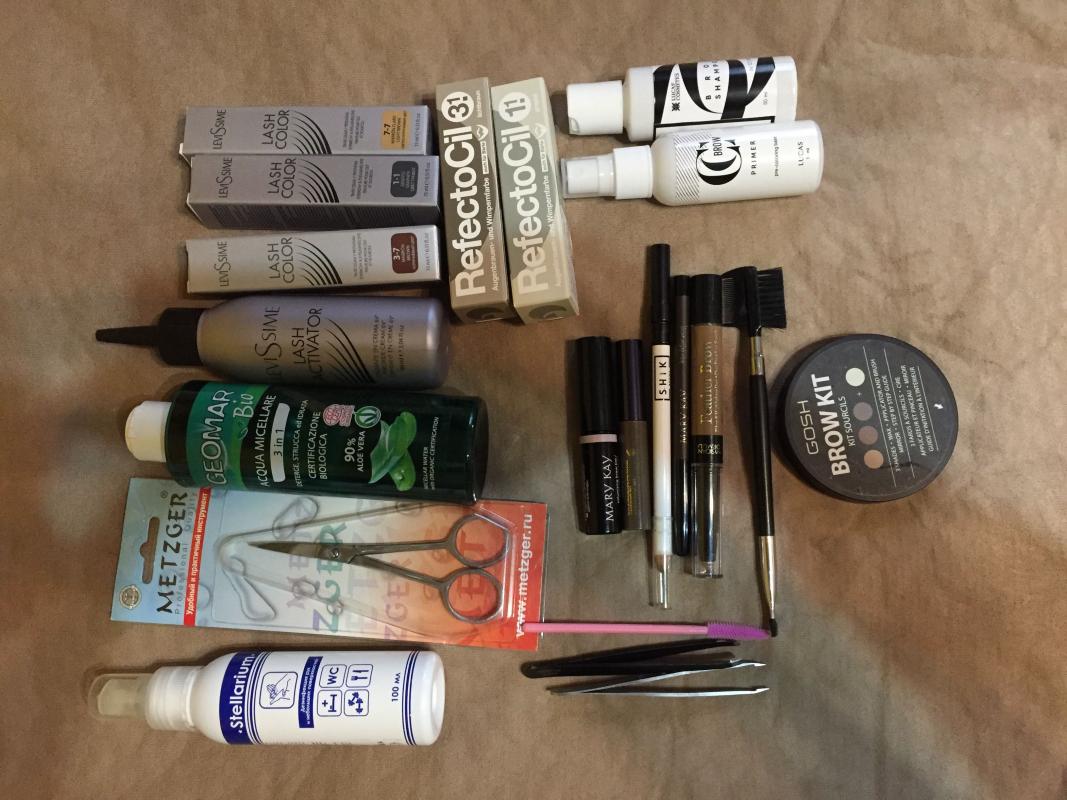The image showcases an array of beauty supplies meticulously arranged on a marble-like background featuring hues of pink and grey. In the top left corner, five small boxes containing hair color tubes are neatly positioned, with two arranged vertically and three horizontally. Adjacent to these boxes, on the right, sit two cylinder-shaped containers lying sideways. Beneath the horizontally positioned hair color tubes, there are a few more cylindrical bottles.

A packaged pair of Metzger-brand scissors is visibly placed right underneath these items. Below the scissors is a small spray bottle, predominantly white with blue accents. To the right of the spray bottle lie several beauty tools, including a pair of tweezers and a pink eyebrow brush. Above these, vertically aligned, are makeup brushes, spot concealer, and a product from Mary Kay. Lastly, situated to their right, is a circular canister labeled as the "Gosh Brow Kit," rounding off the organized collection of beauty essentials.